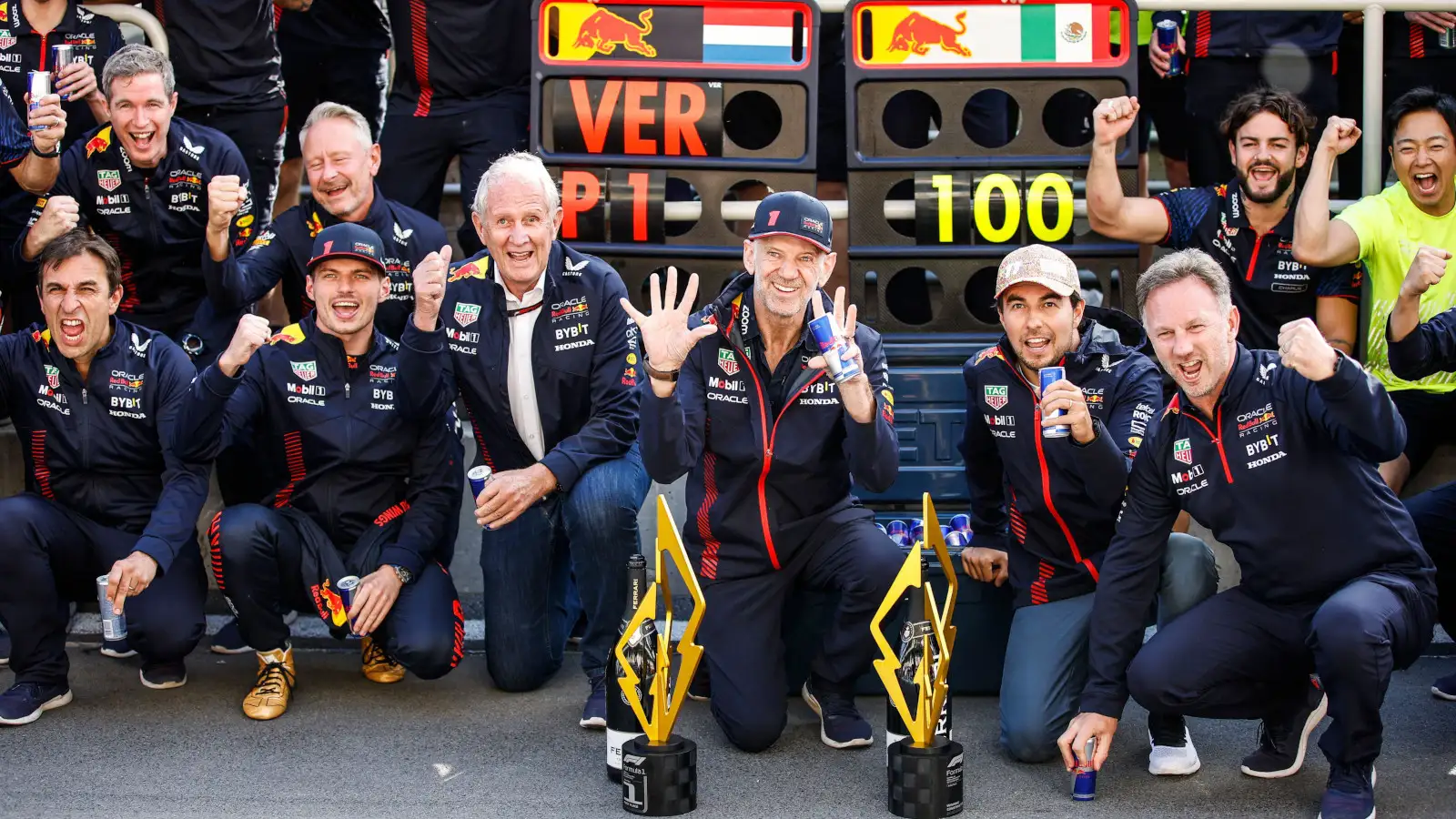This color photograph captures a celebratory moment involving a group of approximately nine men, all attired in matching dark blue uniforms with red zippers. Some of the men are wearing blue hats, while others have white caps or no hats at all. They are positioned low to the ground, either kneeling or propped on one knee, on a gray asphalt street. The men are jubilant, smiling broadly, and many have their fists raised in victory, with the central figure—a white-haired older man—raising all his fingers triumphantly.

In front of the group, prominently displayed on the ground, are two unique trophies. These trophies feature gold or brass-like lightning bolt shapes emerging from black cylindrical bases. Beside the trophies are two giant bottles of champagne, indicating a celebration. Each man is holding a Red Bull energy can, underscoring a sponsorship by the brand.

The background of the photograph includes multiple international flags, notably featuring green, white, and red stripes, akin to the flags of Mexico or Italy. A truck or structure behind the group displays stacks of dark brown cartons with red and yellow stencil lettering, adding to the festive atmosphere.

One individual, distinct from the team, stands at the far right in a yellow shirt, suggesting he is not part of the core team. Clues such as the signage behind them, including "VRP 1" and "100", add context to the sport or event they are celebrating, although the specific sport remains ambiguous. The men’s unified appearance, combined with their exuberant expressions and symbolic trophies, vividly conveys their victorious moment.